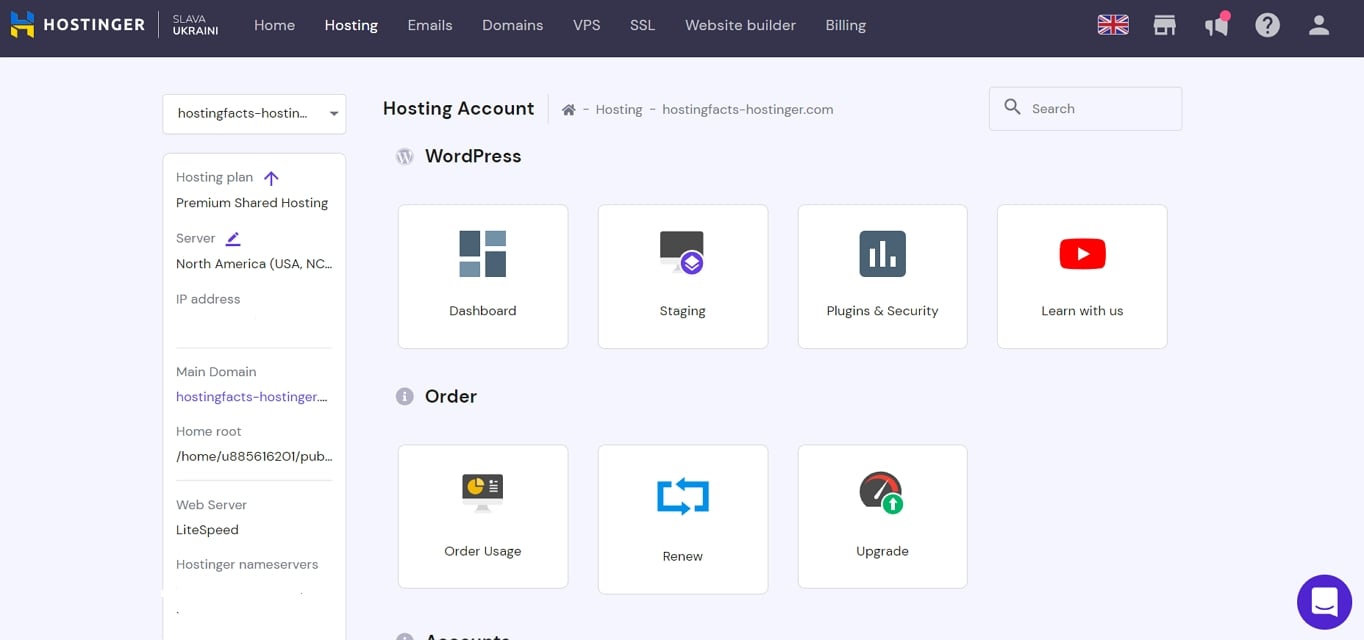The image shows a Hostinger webpage, showcasing their hosting services platform. At the top, the Hostinger logo consists of a blue and yellow 'H', paired with the phrase "Slava Ukraini". The interface includes a navigation bar offering multiple sections: Home, Hosting, Emails, Domains, VPS, SSL, Website Builder, and Billing. There is a prominent United Kingdom flag icon along with several functional icons including a storefront, a notification bell, a question mark, and a user profile outline.

The body of the page is divided into several sections. A main section labeled "Hosting Plan" features a purple upward arrow and highlights "Premium Shared Hosting". This is accompanied by a server icon with a pencil, and details such as the location "North America, USA, NC", as well as an IP address, main domain, home route, and web server information.

The "Hosting Account" section includes a variety of WordPress-related icons. For instance, there is a "Dashboard" icon with multiple windows, a "Staging" icon featuring a computer screen and a purple symbol, and a "Plugins and Security" section represented by a bar graph icon. Additionally, a "Learn With Us" button is displayed alongside a YouTube icon.

Further down, under the "Order" category, options like "Order Usage", "Renew", and "Upgrade" are present. The "Upgrade" section highlights a speedometer icon with a green background and a white upward-facing arrow, signifying performance enhancement.

The majority of the page features a clean, white background, with a darker gray bar at the top containing the main navigation elements in black text.